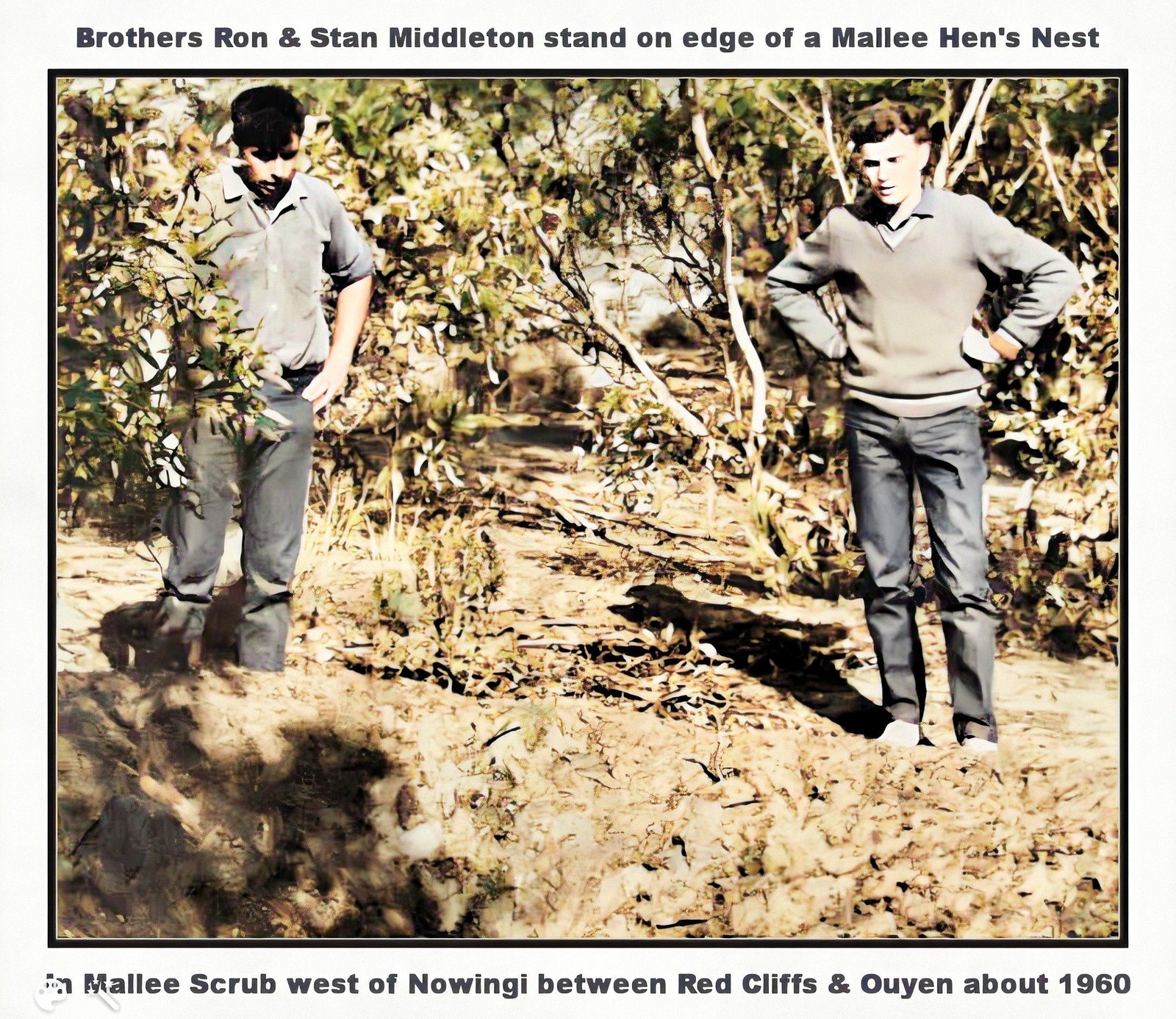This is a colorized photograph from around 1960, depicting two young men named Ron and Stan Middleton standing on the edge of a mallee hen's nest in a mallee scrub west of Nalingi, between Red Cliffs and Ouyen. Both men are wearing light gray sweaters and blue jeans; the man on the left has his sweater rolled up to his elbows and his hands in his pockets, while the man on the right has his sweater hanging normally and his hands on his hips. The background features dulled tones of greenery, with a notable eucalyptus tree and chaotic small bushes. The text above the image reads: "Brothers Ron and Stan Middleton stand on the edge of a mallee hen's nest," and below it says: "In mallee scrub west of Nalingi, between Red Cliffs and Ouyen, about 1960." Despite the image’s apparent AI editing, which gives the people an unusually smooth appearance, the photograph captures a historical and natural setting typical of that era.